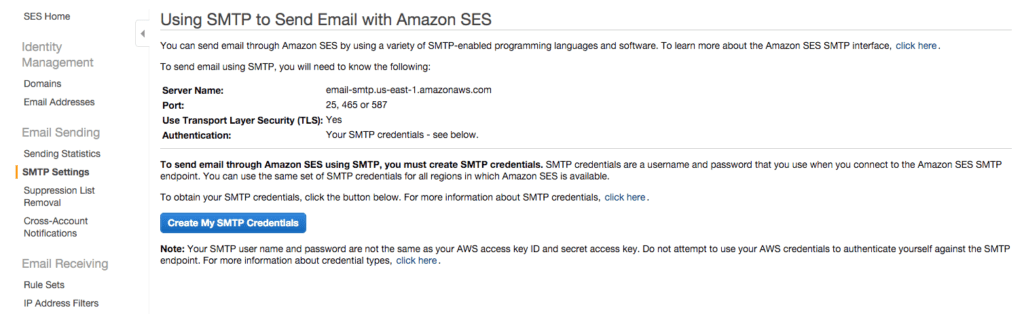A screenshot of a technical interface designed for IT professionals focusing on email configuration through Amazon Simple Email Service (SES). On the left, a navigation pane displays various menu options such as Identity Management, Domains, Email Addresses, Email Sending, SMTP Settings, Suppression List Removal, and Cross-Account Notifications, among others—all relating to email management and configuration.

The main content area on the right is focused on SMTP settings. It provides instructions for sending emails via Amazon SES using various SMTP-enabled programming languages and software. It mentions the necessity to understand specific details such as the server number, name, port, transport layer security, and authentication information. There is a blue button labeled "Create My SMTP Credentials," prompting users to generate the necessary credentials to utilize Amazon SES for email sending. The overall interface is designed to facilitate the setup and management of email services through Amazon's platform, although detailed knowledge of SMTP and related configurations is required for proper operation.